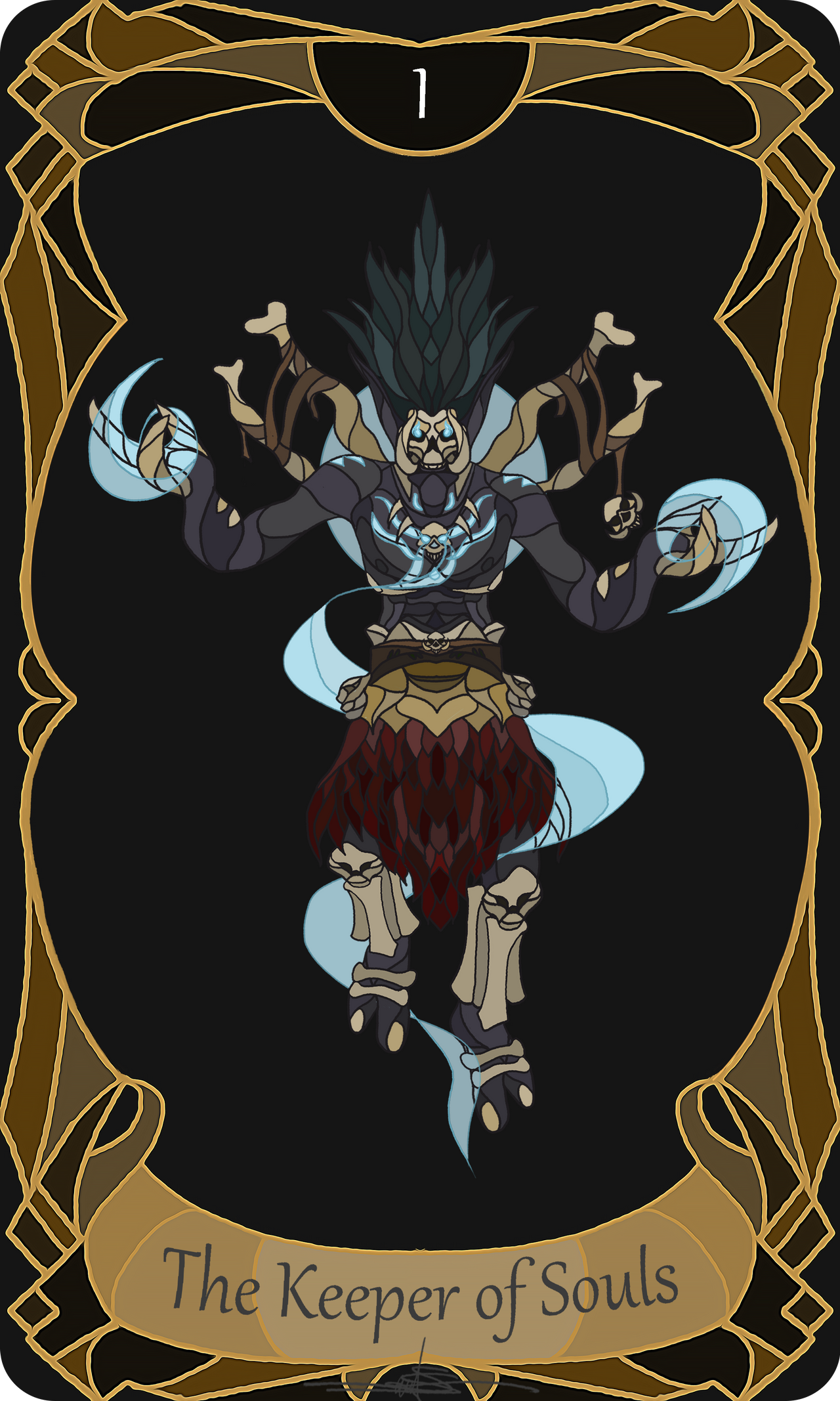The image is a detailed depiction of a tarot card labeled as "The Keeper of Souls," marked with the number 1 at the top center. The background is black, with an intricate frame in gold and bronzish hues surrounding the central figure. At the bottom, there is a tan banner displaying the card's title. 

The central figure is a menacing skeletal being with black skin and striking blue eyes. Its head features a skull-like appearance and long, spiky black hair. The figure's chest showcases a prominent skull, and it has a narrow waist adorned with a red skirt or kilt. Bones and skulls decorate its shin guards and kneecaps, enhancing its fearsome look. 

From the creature's back, two long bones protrude like a grim backpack, resembling femurs. It wears a necklace with a central skull and two fangs on each side. The figure’s hands have claw-like fingers radiating a blue power, which swirls around its form. The entire scene is reminiscent of a dark anime or fantasy design, conjuring an atmosphere of mysticism and dread.